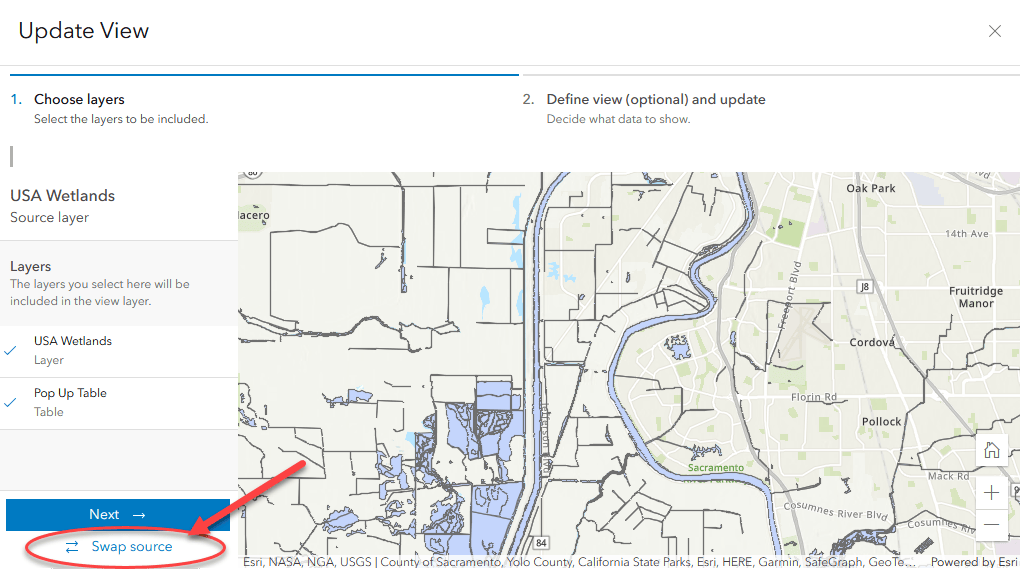This screenshot captures the backend interface for configuring map settings, likely within a mapping or GIS application. Dominating two-thirds of the image is a large, detailed map, though the exact location is not immediately clear. Notably, there is a tag at the bottom of the map that reads "USGS (US Geological Survey), County of Sacramento, California State Parks," indicating that the map pertains to regions within California.

To the left of the map is a vertical menu bar labeled "Choose Layers." At the top of this menu, there is an option to "Update View," followed by the selected "Choose Layers" section. Within this section, the main focus is on "USA Wetlands Source Layer," with additional text explaining that the layers chosen here will be incorporated into the view layer. Currently, both "USA Wetlands" and "Pop-Up Table" options are selected. Just below these selections is a prominent blue "Next" button with an arrow, suggesting a progression to the next step in the settings process.

Further down, there is another button labeled "Swap Source," accompanied by a red circle and arrow deliberately highlighting this option. This indicates the creator’s intention to draw the viewer's attention to the "Swap Source" feature, implying that it’s an important action to take.